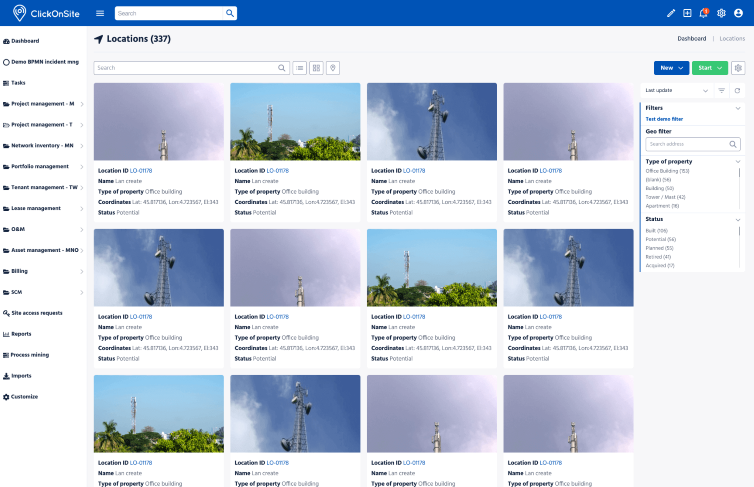**Screenshot of ClickOnSite Web Interface**

The screenshot showcases the user interface of a website called ClickOnSite. In the top left corner, the website's logo "ClickOnSite" is prominently featured, accompanied by a search bar. Below this, along the left-hand column, a detailed navigation menu is visible, listing options such as Dashboard, Demo, BPMN, Incident Map, Tasks, Project Management (with sub-categories M and T), Network Inventory, Portfolio Management, Tenant Management, Lease Management, O&M, Asset Management, Billing, SCM, followed by partially blurry text that appears to read Site Access Request, Reports, Process, more blurry text, Imports, and Customize.

On the right side of the page, there is a gallery of numerous outdoor photographs, predominantly depicting the tops of metal towers. Each photograph is accompanied by details such as Location ID, Name, Type of Property, Coordinates, and Status, with all properties categorized as Office Buildings. The far right column features a set of Filters, beginning with "Type of Property" which has options like Office Building and Apartment. Below this, the Status filter is present, although partially blurry, possibly including headers like Potential, Planned, among others that are illegible due to poor clarity.